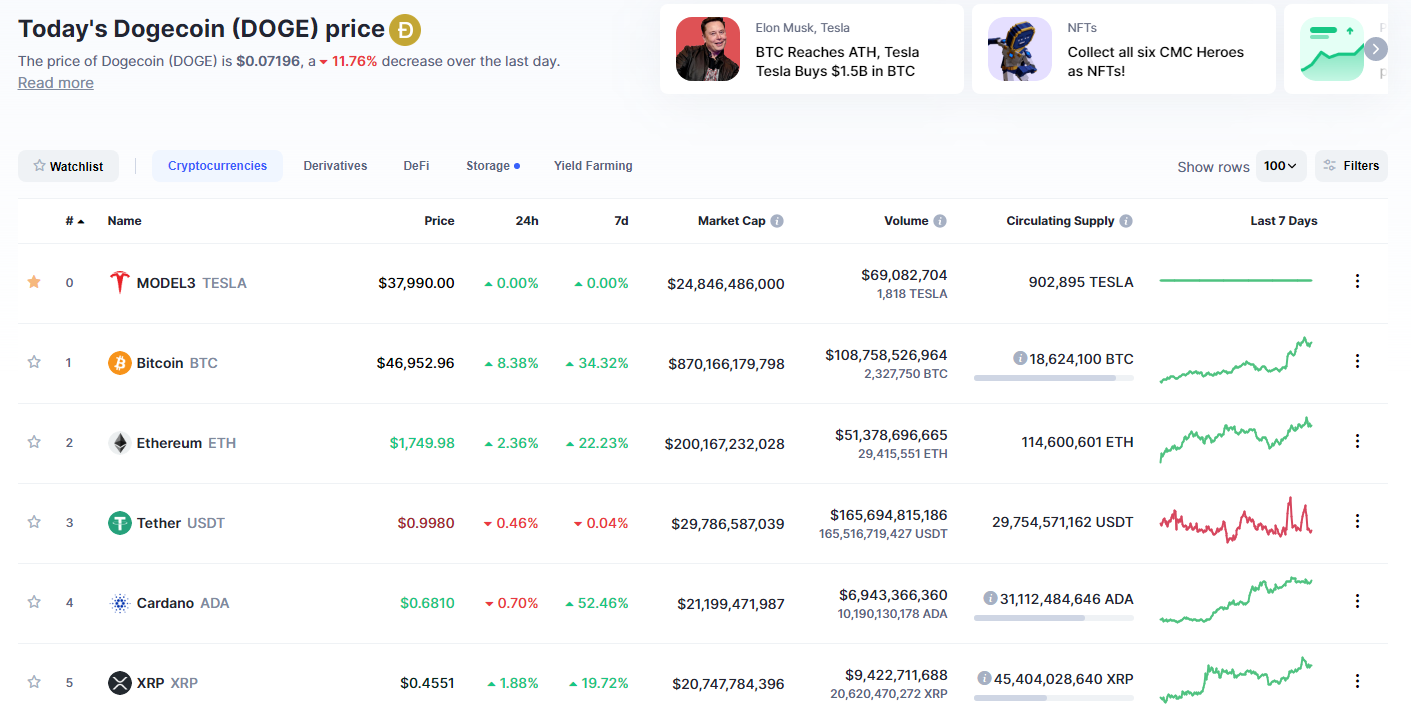The image provides detailed information on the current price of Dogecoin, marked prominently at the top left with the header "Today's Dogecoin." Directly beneath this, it reaffirms in parentheses with "DOGE PRICES." The current price of Dogecoin is listed at $0.07196, repeated twice for emphasis. Additionally, a red downward arrow indicates an 11.76% decrease over the past day, signifying a decline in value. Below this information, a "Read More" button is underlined, suggesting further details are available upon clicking.

The image also features several tabs along the top, but some are partially cut off. The visible tabs include "Watchlist," "Cryptocurrencies," and possibly "Derivatives." The remaining tabs, "Storage" and "Yield Farming," are more clearly visible towards the end.

Further down the image, there is a list of various assets and their corresponding prices. This list includes Model 3 Tesla, Bitcoin (BTC), Ethereum (ETH), Tether (USDT), Cardano (ADA), and XRP, though specific prices for these assets are not clearly mentioned in the caption.